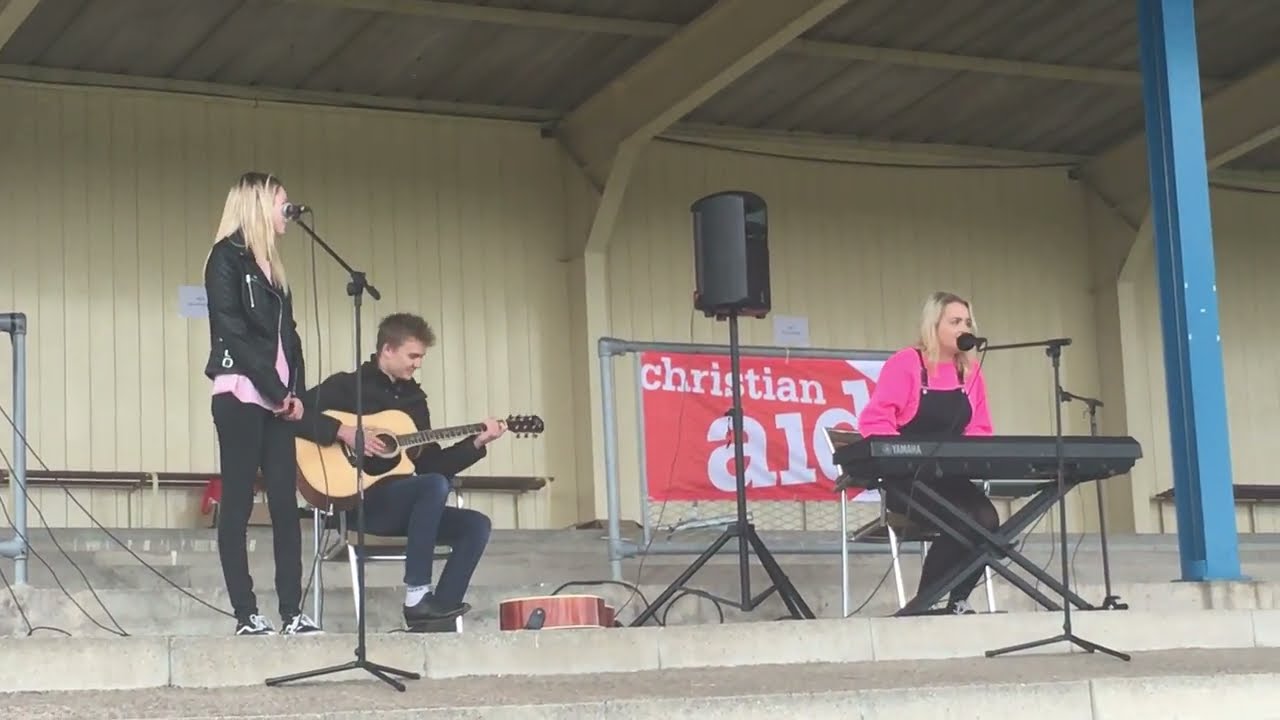The photograph captures a vibrant outdoor stage setup where a young, dynamic trio of musicians is performing. Central to the scene is a male guitarist dressed in black, seated and strumming an acoustic guitar. To his left stands a young blonde woman, exuding energy as she sings into a microphone. She wears a pink shirt, a blue jacket, dark blue or black pants, and black sneakers. To his right, another blonde woman, also in a pink shirt but with a white vest, is seated at a black Yamaha keyboard, singing into a microphone. Behind her, a prominent sign with the text "Christian Aid" set against a red background provides context for the event, suggesting a charitable performance. The stage is framed by a brown wall, adding to the setting's warm, inviting atmosphere. A large speaker on a tripod stands to the right of the guitarist, ensuring their music reaches the audience. The band appears to be performing during the day, possibly on the steps of a building that resembles a stadium or auditorium, looking slightly to the right as if engaging with an audience gathered there. The scene is brightly lit, highlighting the lively spirit of their performance.